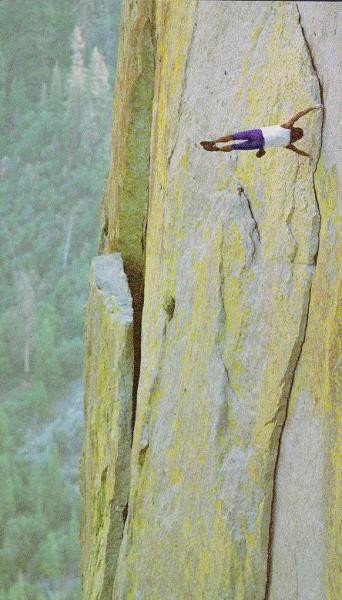A man is captured performing a handstand on a rugged, high rock formation under a grayish-blue sky dotted with clouds. The image, taken from a unique sideways perspective, highlights the contrast between the bright, yellow-tinged rocks and the blue sky. The man is dressed in a white tank top, purple knee-length shorts, and black shoes. He wears white gloves and appears to have a cell phone holder attached to his belt. The rocky surface, speckled with sharp pieces and occasional patches of green leaves, adds an element of danger and adventure to the scene. The man’s poised handstand against the dramatic sky backdrop makes for a striking and potentially social media-worthy photograph.